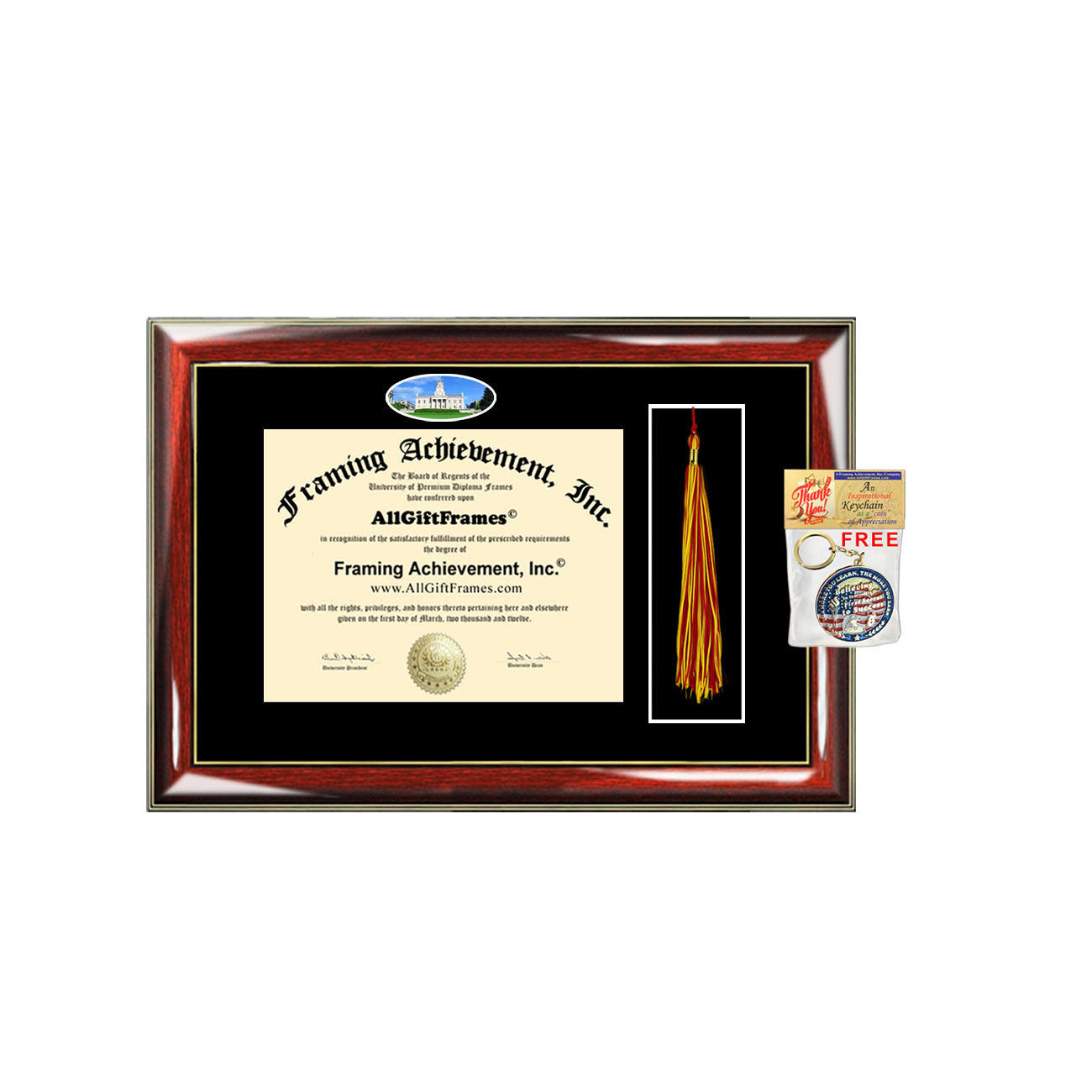This is a horizontally aligned rectangular frame with a mix of materials; the outer frame appears to be thin, silver metal while the inner frame is made of cherry wood. Inside the frame, there is a black backing with a square section in a light tan color, holding a detailed certificate. The top of the certificate features an oval graphic displaying a house, a grassy area, and a tall building against the sky. The main text of the certificate, titled "Framing Achievement, Inc.," reads that the Board of Regents of the University of Premium Diploma Framers has awarded the degree of Framing Achievement to all gift frames in recognition of fulfilling the necessary requirements. Below is the URL, www.allgiftframes.com, and fine print detailing rights and privileges, dated March 1, 2008. A gold seal and signatures are embossed at the bottom. To the right of the diploma hangs a gold tassel, and adjacent to it is a small package with a keychain featuring an American flag design and labeled "Free." The diploma is bordered by a brown frame, enhancing its presentation.